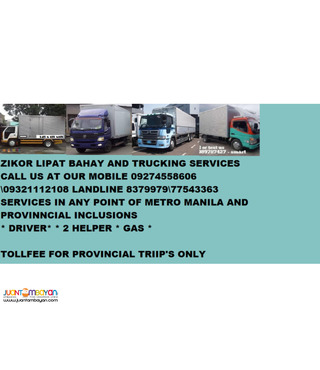A rectangular screenshot with a mint green background and bold black text is depicted. The text prominently reads, "Zecor Lipat Bahay and Trucking Services." Contact details are provided: "Call us at our mobile 092-745-58606, landline 837-9979, 775-433-63." Below, it states, "Services to any point of Metro Manila and Provincial Inclusions." Additional details specify: "Driver, helper, and gas fees," with a note in the lower left corner that says, "Toll fee for provincial trips only." In the upper left corner, there is a color photograph showing multiple trucks.